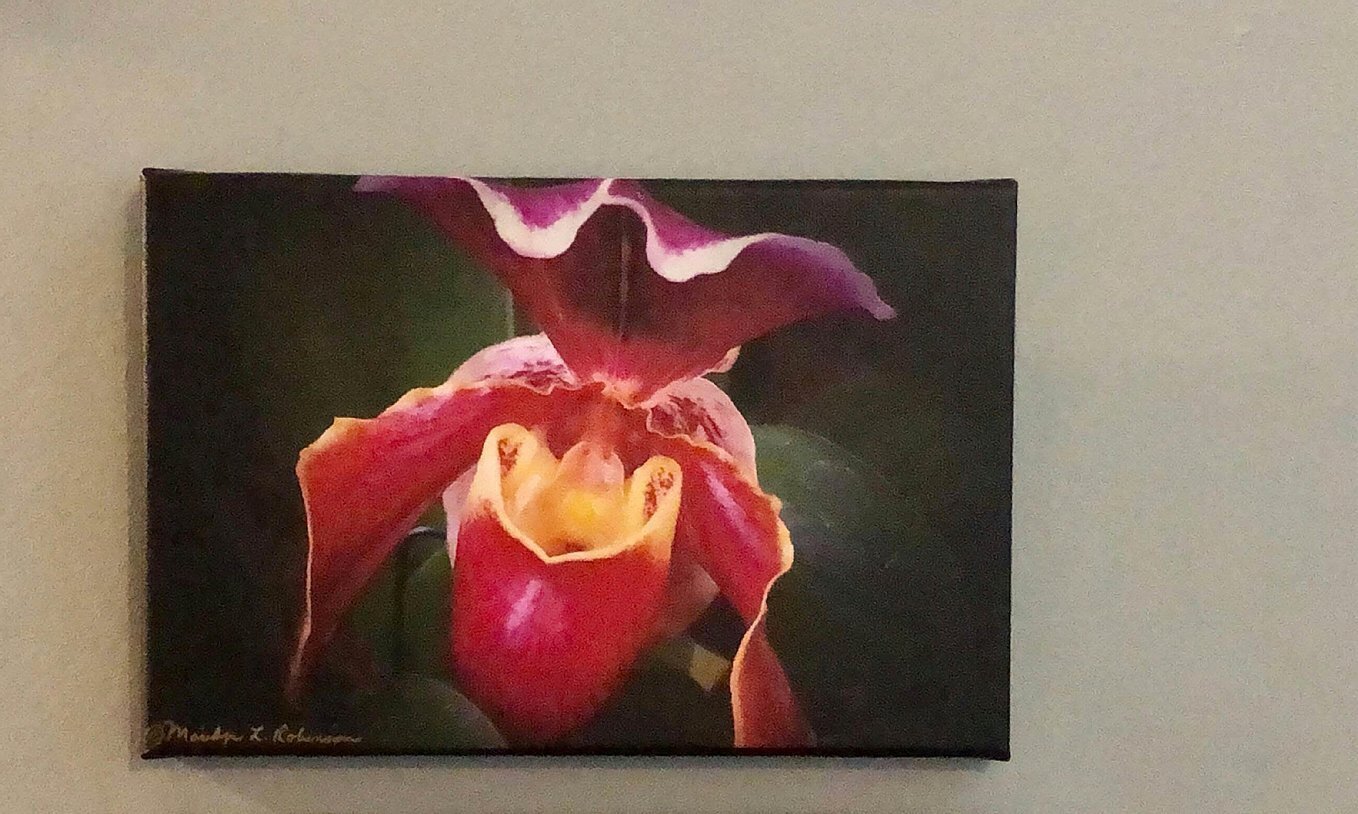The image shows a painting mounted on canvas and hung against a gray-beige wall. The artwork, a close-up print of a flower, features petals in shades of pink and purple, with rich yellow accents in the flower's center. The petals appear flowy and dynamic, almost as if they're emerging from the bud, surrounded by subtle, blurred green leaves in the background. The flower, possibly an orchid, displays various tones and gives the impression of multiple flowers intertwined. The artist's signature is located in the bottom left corner of the frame, though it is not clearly legible.